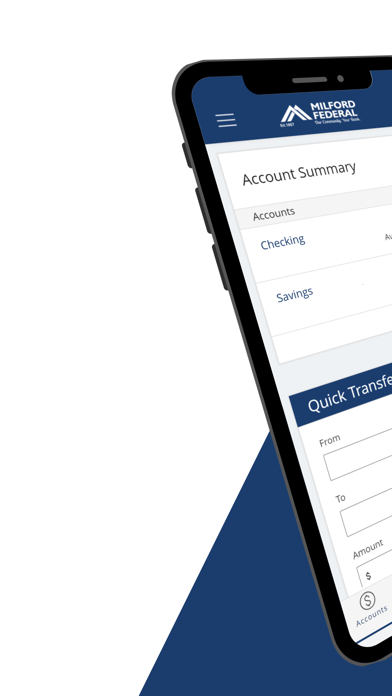The image appears to be a digitally rendered advertisement featuring a partial view of a black cell phone with a notably thick bezel and an upper notch. The screen displays the website of "Milford Federal," characterized by a navy bar at the top containing white lines for navigation. The screen content beneath shows a white background with clear black and blue text outlining account details: "Account Summary," "Accounts," "Checking," and "Savings." A prominent navy header highlights "Quick Transfers," including fields for "From," "To," and "Amount," denoted by an icon of a circle and a dollar sign. 

On the side of the cell phone, three buttons are visible. Behind the phone, there's a pixelated navy triangle adding to the digital aesthetic of the image. The overall image quality is high, with bold and legible fonts. The design is clean, straightforward, and effectively simulates the cell phone's interface without additional elements to distract from the focal point.